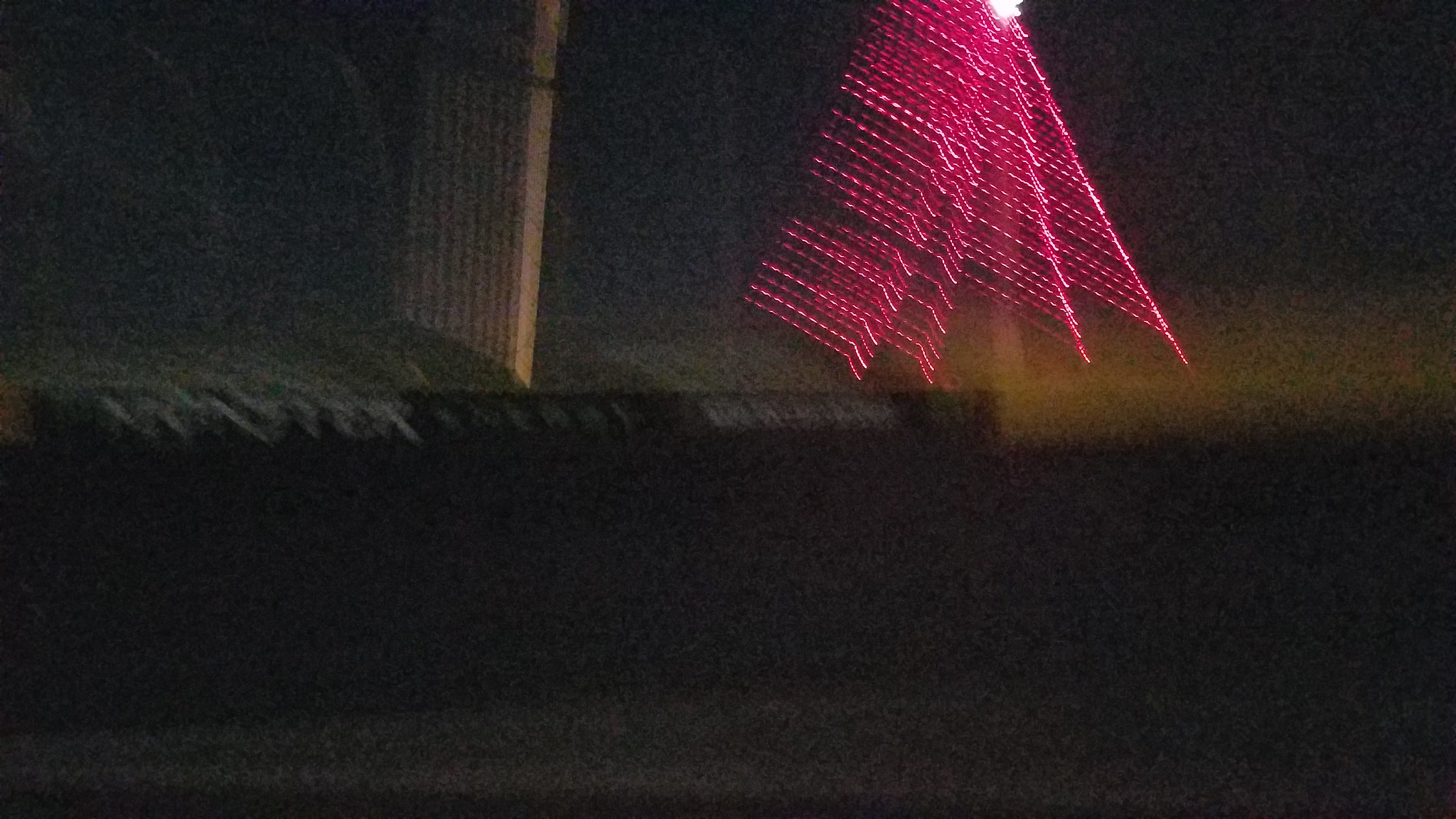This extremely blurry image presents a predominantly black background with indistinct light gray or dark gray areas at the bottom left. A broad brown streak spans horizontally across the top portion, almost resembling a shelf. Notably, about a third into the image from the left side, there is an indistinct vertical brown blur, while two-thirds in, a vertical magenta blur appears, somewhat reminiscent of a tree formation. Contributing to the chaotic composition, a bright white light emerges from the top, extending downward towards a brown blur located from the right side to the magenta formation. The lower foreground is shrouded in darkness. Upon closer inspection, multiple pink dots, suggestive of lights, cascade up and down, adding to the frenzied motion hinted at by these blurred elements, particularly the cluster of lights creating a ripple or dotted effect akin to lightsabers in motion.